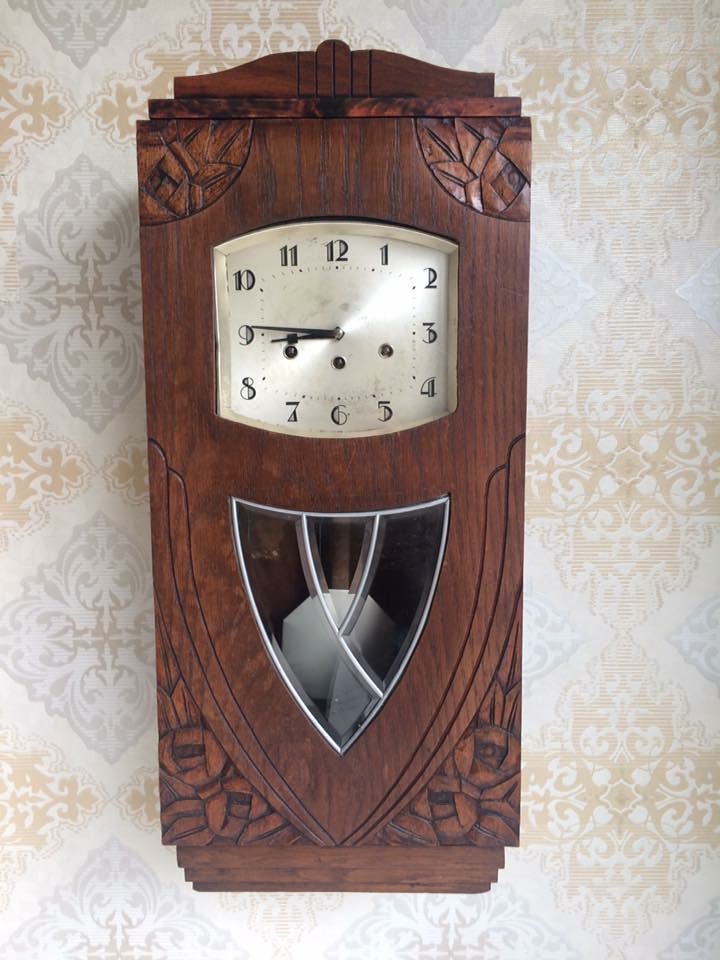The image showcases a wall-mounted clock set against a beautifully adorned wallpaper. The wallpaper features a lustrous silver and white backdrop, intricately designed with a golden floral motif arranged in a diamond pattern. The clock itself is crafted from dark-stained wood and has a distinctive rectangular shape, hanging vertically on the wall. Each corner of the clock is embellished with elaborate floral carvings, adding an ornate touch.

The clock face has a pearlescent white hue, adorned with black numerals and black hour and minute hands. Below the main dial are three small dark circles whose functions are not visible. Additionally, a chime mechanism is housed within an inverted triangular glass compartment at the base of the clock. This glass compartment is framed with metal and features internal metal crossbars. The chime inside appears to be a round piece with a white or silver finish, contributing to the clock’s elegant and timeless appearance.